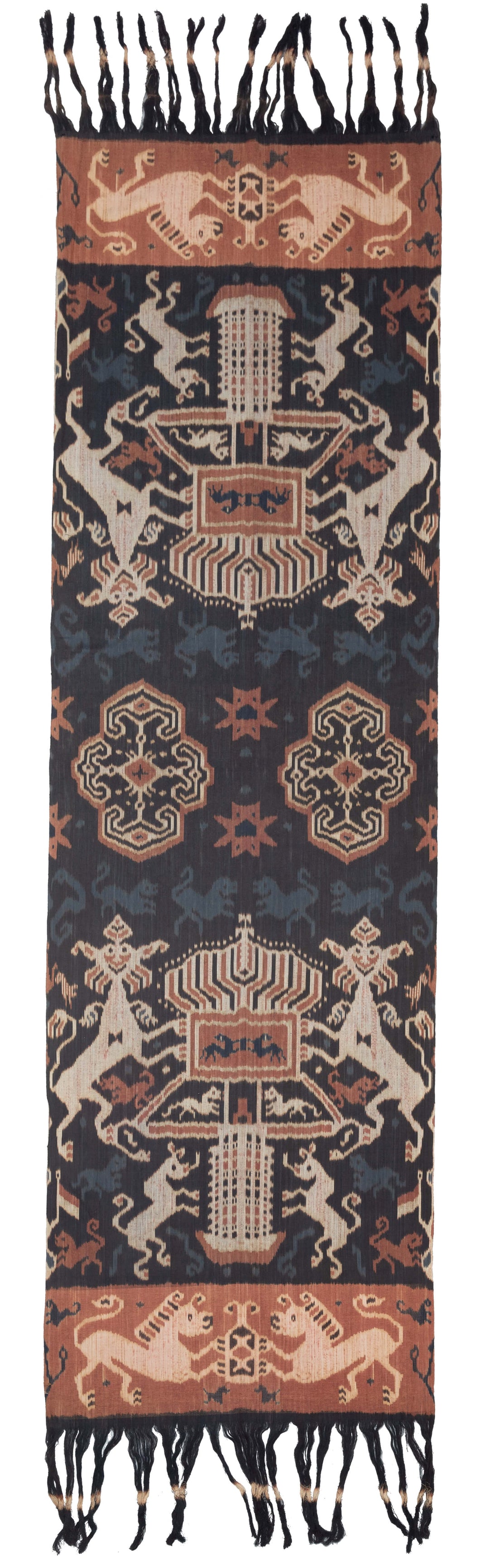This image depicts a long, narrow runner-style rug, possibly of Middle Eastern or Asian origin, laid out from a bird's-eye view against a completely white background. The rug features intricate designs, including stylized animals such as horses and dogs with peculiar faces, along with various emblems and shapes that might suggest stars or temples. The dominant colors are shades of blue, brown, tan, white, rust red, and black. The rug also has black tassels at both ends, contributing to its vintage appearance. The detailed patterns and pictorial elements along the runner make it a distinctive and eye-catching piece, suitable for floor placement in a hallway or as a decorative table runner.